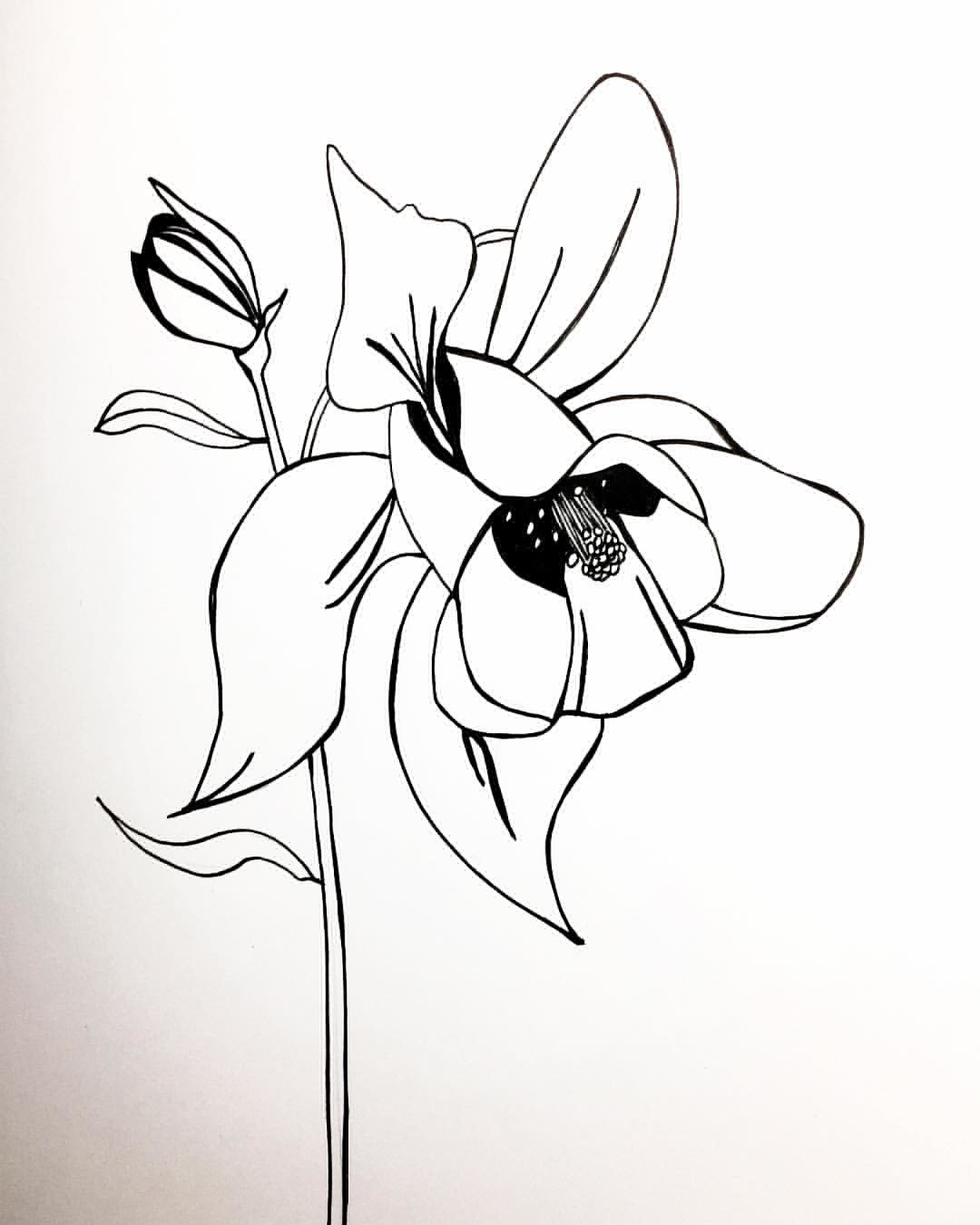This black and white sketch features a detailed depiction of a lily flower and its bud. The drawing showcases a lily with partially open petals, where the outer petals are spread out while the inner petals are yet to unfurl, elegantly hanging down towards the center. The artist has used solid black shading in the middle of the flower to create depth and contrast. Adjacent to the open lily is a tightly closed lily bud, indicating that it has more time before it blossoms. The composition is anchored by a very long stem that splits into two parts, one leading to the open flower and the other to the bud. Accompanying the flowers are small, pointed leaves that extend outward from the stem, adding to the intricate detailing of the piece.